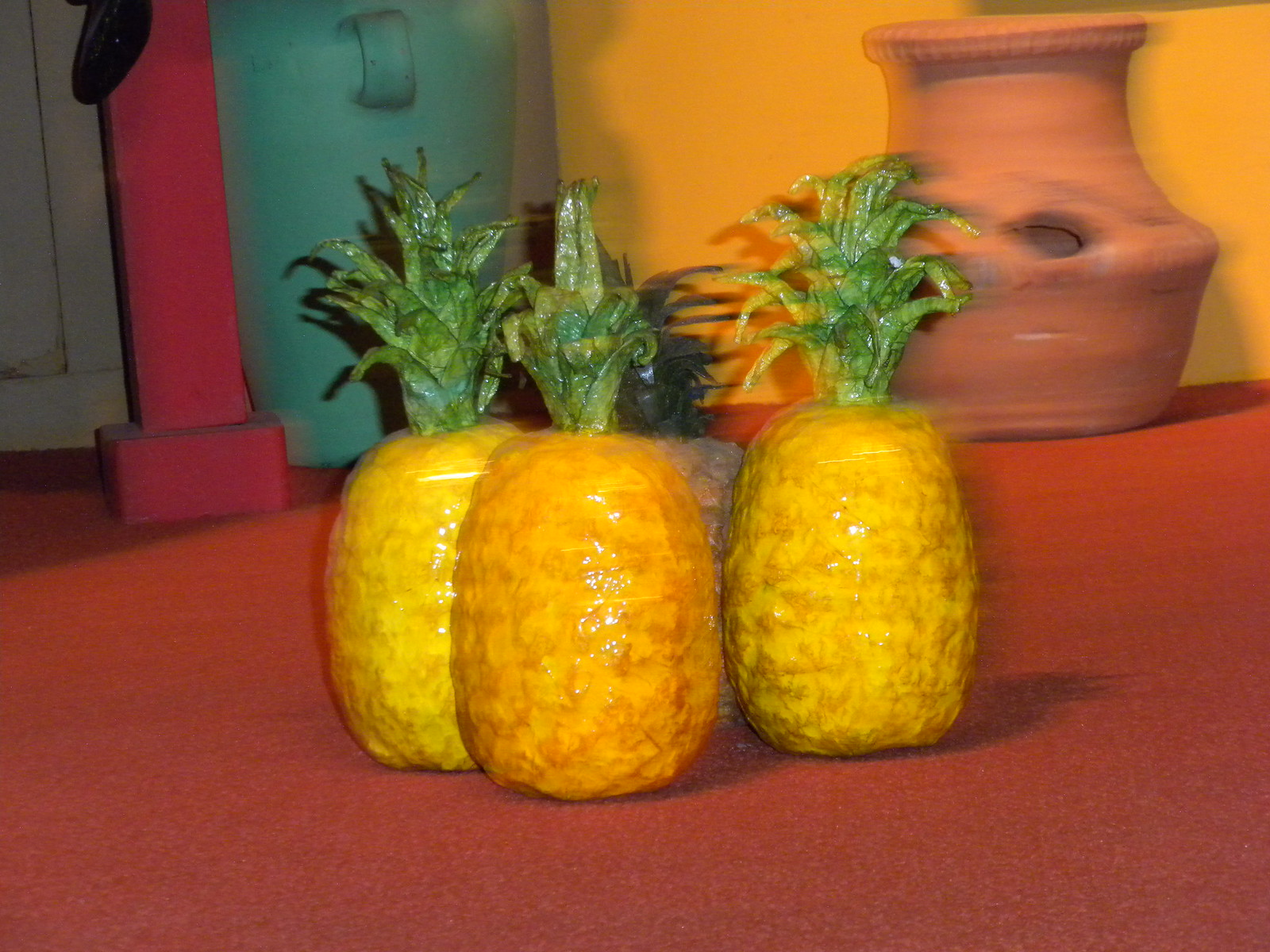This photograph, slightly blurred but mainly in focus, captures a vivid indoor scene with striking details. Set against a vibrant backdrop, the rear wall features a bright orange hue transitioning to a mustard yellow toward the right. Prominently displayed near the back is a blue cylindrical jug with a handle, juxtaposed with a large terracotta clay urn, which has a noticeable hole in it. Adjacent to this is a rectangular red wooden column partially visible. The floor is covered with a bright red carpet, on which four pineapples rest. Three of these pineapples are a shiny yellow with glossy green leaves on top, wrapped in bubble wrap, giving them a slightly unreal, sculptural appearance. A fourth pineapple, partially concealed by the others, appears to be decayed with darker, almost black leaves and a duller body, suggesting it might also be a decorative piece. The setting blends an array of colors and textures, making the scene both visually stimulating and intriguing.